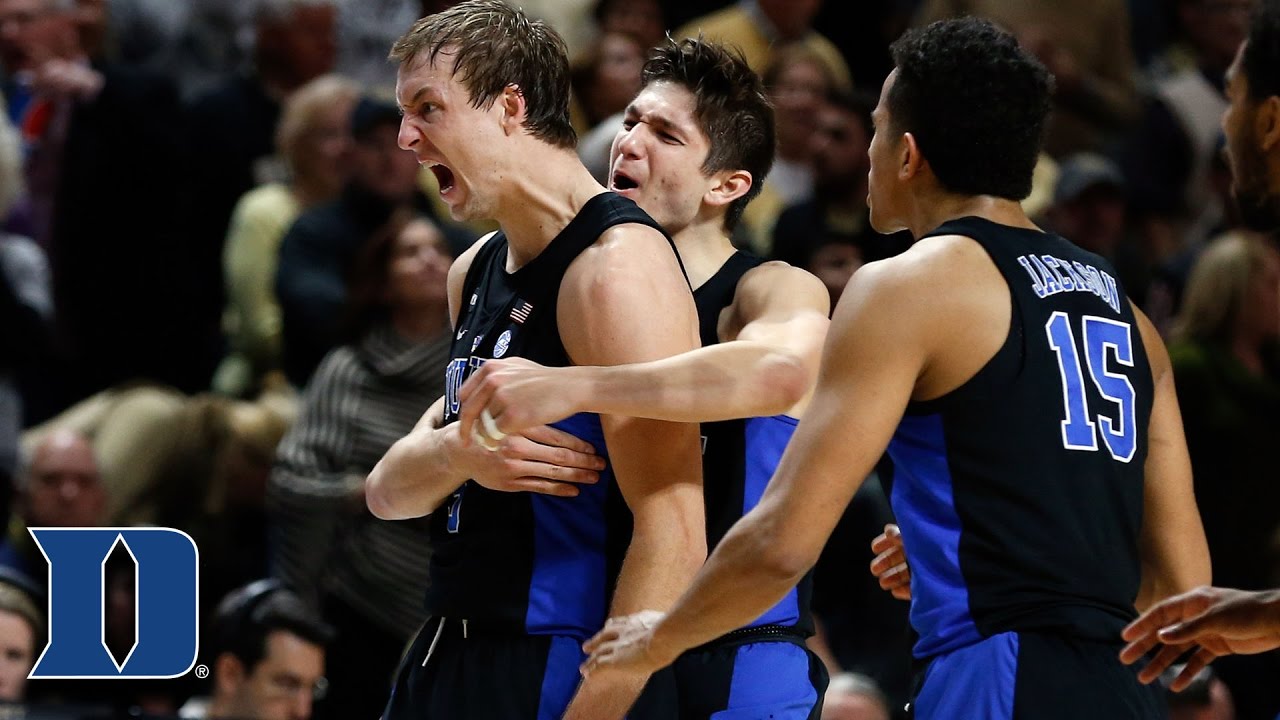The photograph captures a thrilling moment during a Duke University men's basketball game. Three players, sporting black and royal blue jerseys with blue accents on the sides, are the central focus. The player in the middle, with short brown hair just past his ears, appears to be yelling in sheer excitement or celebration, his mouth wide open. Behind him, another muscular teammate is embracing him in a backwards hug, wrapping his left arm around the yelling player’s chest and bringing his right arm around in a comforting gesture. Approaching them from the right is a third player, whose face is partially obscured, but his jersey is clearly visible, displaying the number 15 and the last name "Jackson." The iconic blue 'D' logo of Duke University is prominent in the bottom left corner of the image. The background reveals a muted crowd, their faces blurred, emphasizing the intensity and emotion of the players in the foreground.